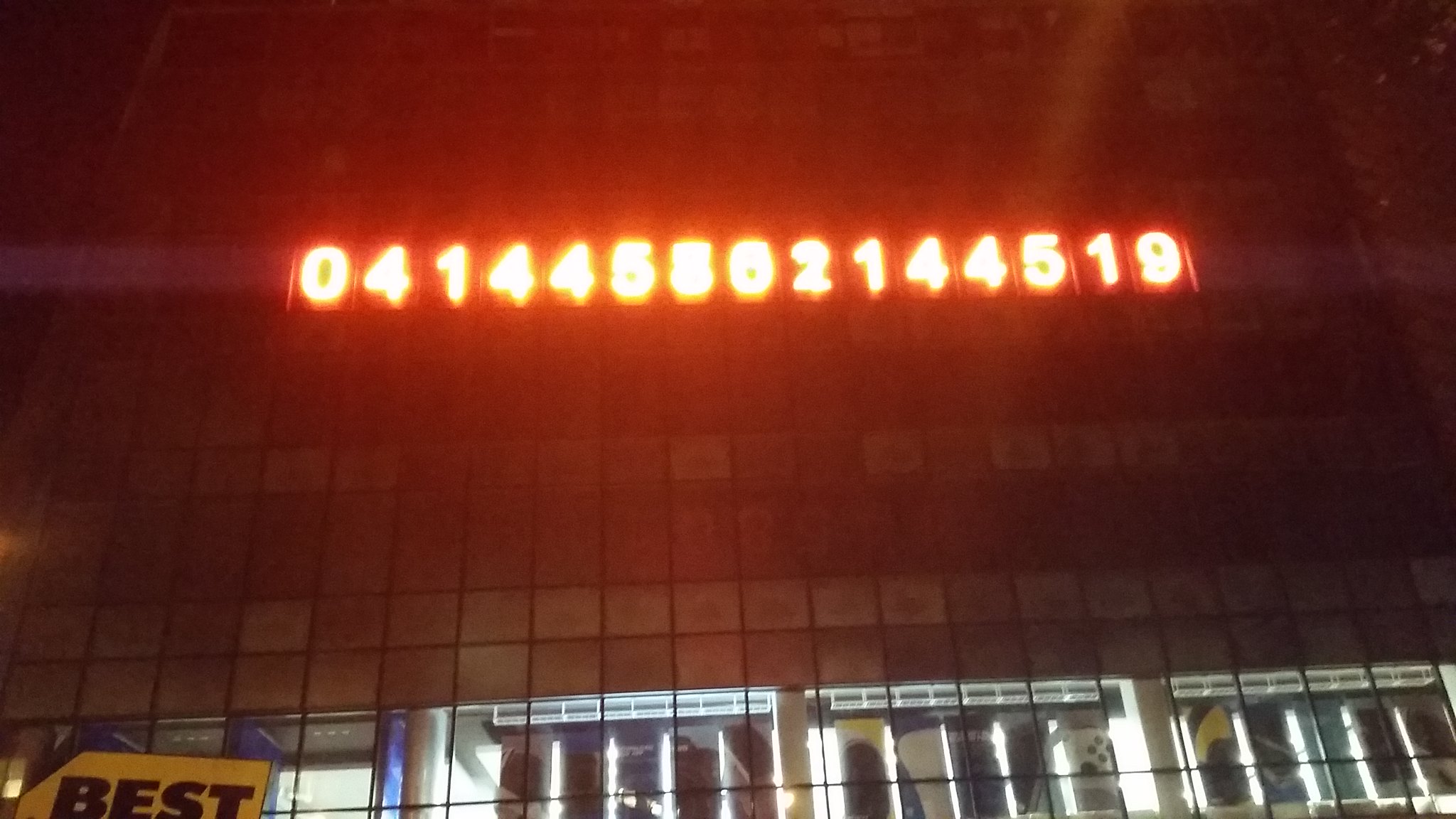The image depicts the facade of a modern building adorned with an extensive digital display at the top, showcasing a sequence of red LED numbers: 0, 0, 1, 4, 4, 5, 5, 0, 2, 1, 4, 4, 5, 1, 9. Beneath this numerical display, the building features multiple rectangular windows aligned in a grid pattern, reminiscent of a typical, contemporary architectural design. The windows have black lines framing the glass panes, which are further divided by slender horizontal and vertical mullions. A sign announcing "Obama says Best Buy" is prominently displayed, suggesting a promotion or endorsement. On the right side of the image, additional windows can be seen with light streaming through, indicating interior illumination. This combination of the digital display, structured grid of windows, and penetrating light contributes to a visually engaging urban scene.